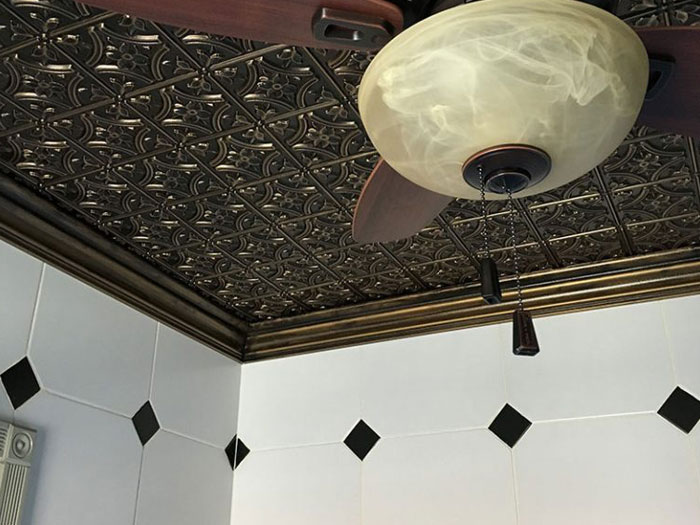The image captures the ceiling and upper wall of an interior space, featuring a decorative tin ceiling composed of square tiles with intricate, floral, metal designs. The tiles exhibit a mix of bronzish and greyish hues, accentuated by a pattern that includes interlocking dark blackish-brown circular shapes. The ceiling seamlessly transitions into the wall with a brownish trim. Below the ceiling, the upper part of the white wall is adorned with a geometric design of black squares and diamond shapes formed by the alignment of black triangle corners in adjacent tiles.

Prominently displayed in the image is a ceiling fan with brown, cherry wood-like blades. Attached to the fan is a light fixture with a dome-shaped, pearly white, marble-like design, embellished with wisp-like patterns and a central dark circular disc. The fan and light fixture can be controlled via two pull chains that hang down, designed for adjusting the light and fan speed.